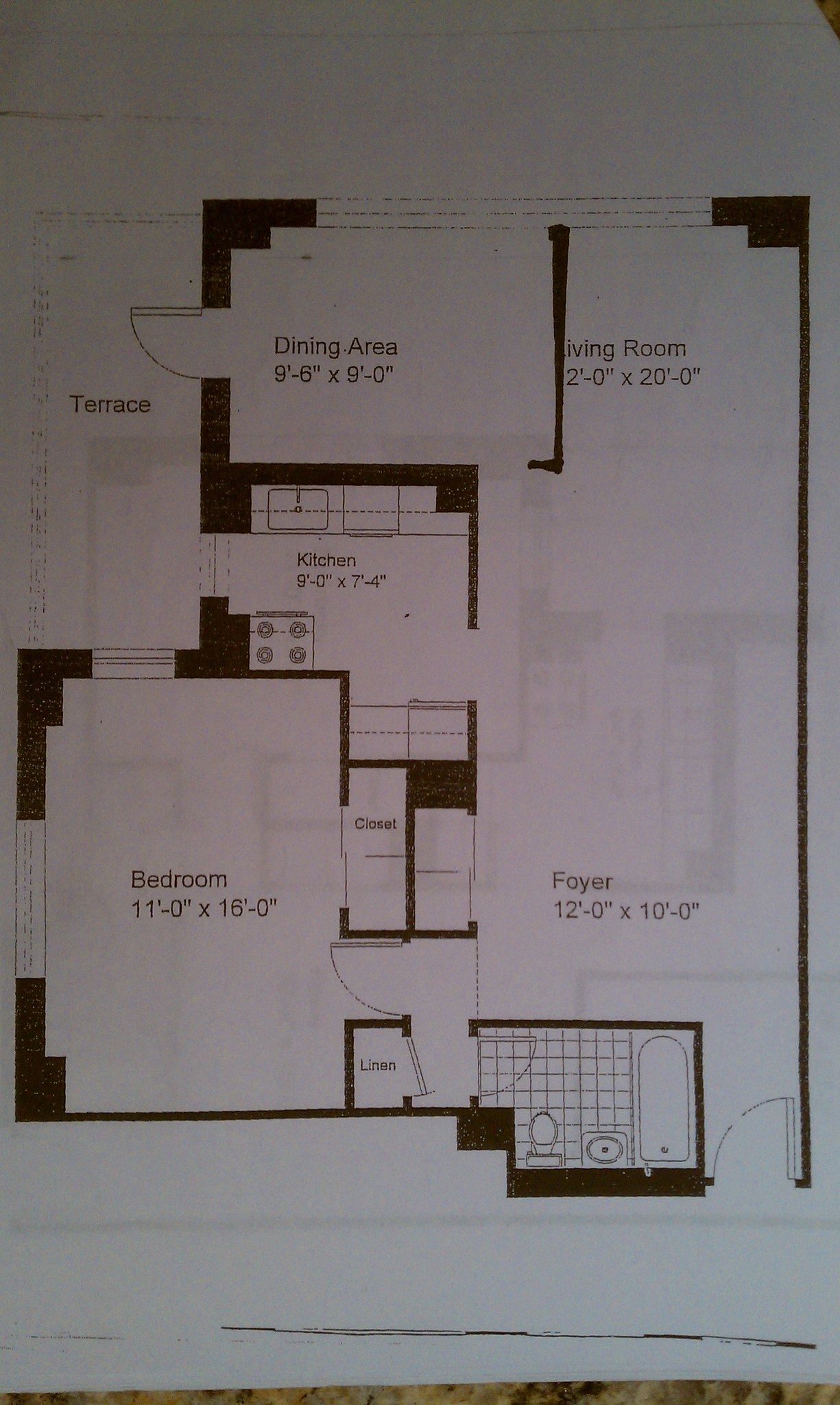A detailed black-and-white photocopy of an apartment floor plan is presented on a plain piece of paper. The most expansive area, occupying the right half of the layout, is the combined living room and foyer. In contrast, the upper left-hand corner features the dining area, which has direct access to a terrace via a doorway. Situated below the dining area is the kitchen, while directly beneath the kitchen, there is a spacious bedroom equipped with a substantial closet and a linen closet. The bottom section of the floor plan is dedicated to the bathroom. Specific measurements for each room are included: the dining area measures 9'6" x 9'0", the kitchen is 9'0" x 7'4", and the bedroom spans 11'0" x 16'0".